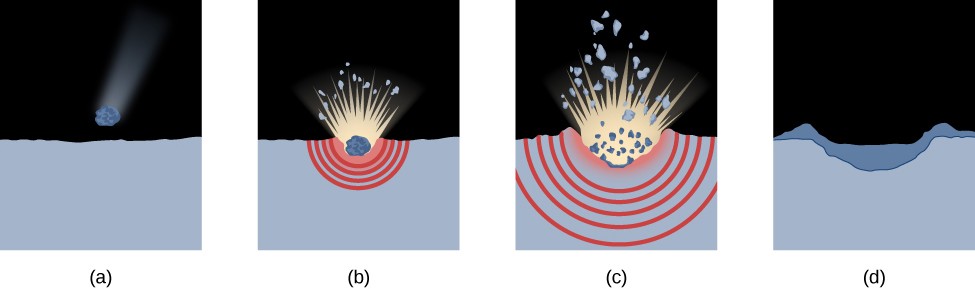The image is a detailed, artistic sequence showing the impact of an asteroid or comet on a surface, possibly the Moon. It consists of four illustrations labeled A through D on a white background with black text. 

- Illustration A depicts a celestial blue rock with a white streak in the sky, rapidly descending towards the ground. The sky is black, and the ground has a bluish hue.

- In Illustration B, the asteroid impacts the landmass, creating a small yellow explosion and generating red concentric semicircles in the ground, indicating shock waves.

- Illustration C shows the asteroid breaking apart into numerous fragments, with the red shock waves spreading further.

- Illustration D reveals the aftermath, displaying a crater left by the impact with no visible remnants of the asteroid or shock waves.

This sequence effectively conveys the progression from descent and impact to explosion and aftermath, highlighting the dramatic effects of such an event.